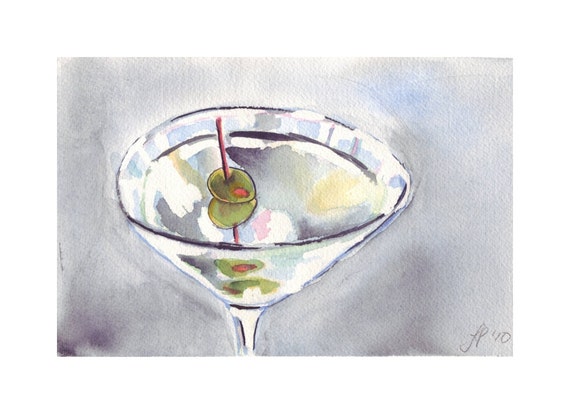This watercolor painting depicts a martini glass set against a predominantly gray background, accented with subtle hues of blue and purple. The center of the composition features the top portion and a partial stem of the martini glass, which is primarily rendered in whites, grays, and blues to convey the transparency of the glass. A black swirl inside the glass indicates the liquid level, adding depth and dimension with darker gray tones. A vibrant red stir stick pierces through two green olives, with the front olive showcasing a distinct red pimento. The liquid within the glass is a pastel blend of gray, purple, light blue, and hints of orange and pink, adding a delicate touch to the otherwise subdued palette. The painting captures the reflective quality of the glass and the olives' placement, suggesting a soft and elegant ambiance.